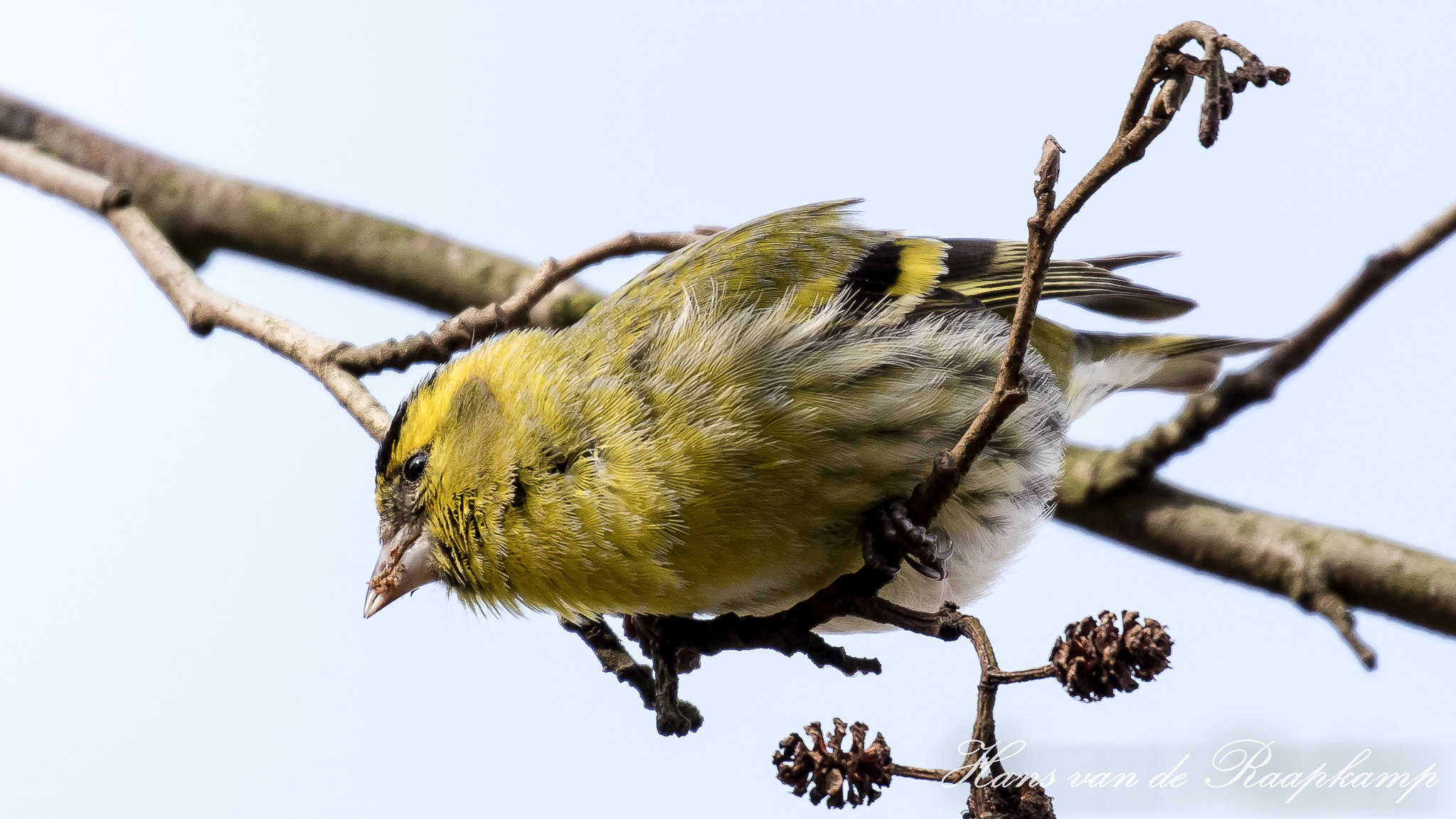In the photograph, a small, fluffy bird, possibly a black-capped chickadee, is perched on a tiny brown twig that juts out from a larger branch. This bird, which looks like it would fit comfortably in the palm of your hand, features a striking mix of colors: its head, chest, and feathers exhibit a blend of yellow and brownish-black hues, while its wings are decorated with alternating black, yellow, and brown stripes. The bird's tail and belly are predominantly white streaked with brown. 

It has a pointed gray beak, black eyes, a small black spot on the top of its head, and black feet gripping the twig. The larger branch, from which the twig extends, diagonally bisects the photograph, stretching from the top left corner to the bottom right and is adorned with small pine cone-like seed pods. All this is set against a flawless light blue sky, devoid of clouds, creating a serene backdrop. A watermark in the corner reads "Hans van der Praakamp," likely indicating the photographer's name. The bird is captured facing slightly downward to the left, with its wings softly cupped to its sides, appearing tranquil in its natural setting.